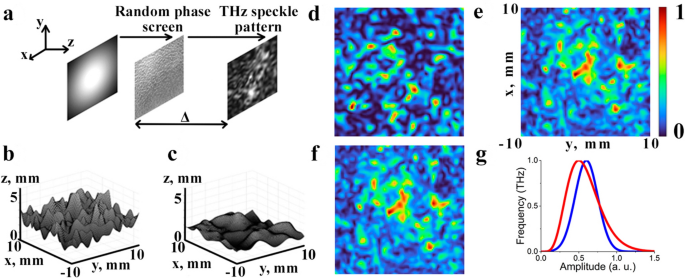The image is a large, rectangular scientific diagram comprising eight different components labeled A through G. Label A features a black-and-white image with black lettering, showcasing a random phase screen THZ speckle pattern, with arrows pointing to three images of squares. Labels B and C include graphs depicting measurements, while Labels D, E, and F display squares filled with colorized pixels. These squares illustrate infrared heat patterns with a blue background interspersed with light yellow, red, and green specks. Label G is a bar graph, marked with "frequency THZ" along the vertical axis and "amplitude" along the horizontal axis, featuring red and blue spiked lines. The diagram collectively visualizes various aspects of frequency, amplitude, and thermal imagery through different graphical representations.